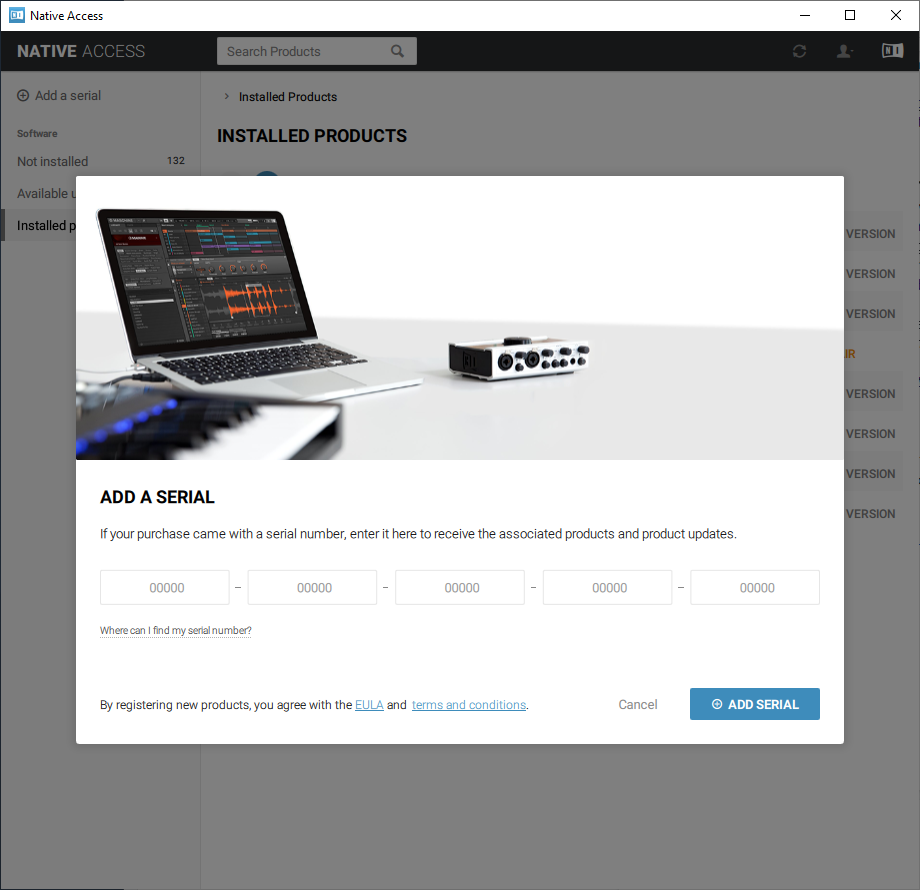The image is a square screenshot featuring a central white pop-up box against a translucent gray backdrop, allowing partial readability of the background text. The upper left corner of the gray background displays "Native Access" in a plain font, while the upper right corner hosts three icons for minimizing, enlarging, and closing the window.

The pop-up box showcases an image of a laptop displaying a music program alongside a segment of a keyboard and an electronic device. Below the image, the text "Add a Serial" indicates that users should enter a provided serial number to access associated products and updates. The serial number entry area consists of five sequential input boxes. At the lower right corner of the pop-up, a blue "Add Serial" button is prominently displayed.

On the lower-left side of the pop-up box, the text guide "Where can I find my serial number?" is followed by information about registration conditions, mentioning EULA and terms and conditions, which are hyperlinked in blue.

In the background, the main window shows a section for installed products under a black header with another "Native Access" title and a search bar. The header also features three icons on the right side, likely for navigation or settings.